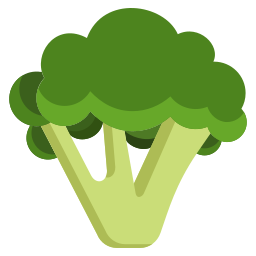This image is a simple, detailed illustration of a head of broccoli set against a plain white background, highlighting its intricate details with no light source or shadows. The broccoli features a light yellowish-green stem that branches into three curved stalks. Each stalk supports a puffy cluster of florets, blending from light green at the base to darker green at the top, with the darkest shades at the back, suggesting depth. The broccoli is rendered in a flat color style with subtle curved edges and olive-green shading around the stem, enhancing its dimensionality. The florets are intricately depicted, with a large, dark green floret in the foreground and circles of darker green suggesting additional florets in the background. This appears to be a clip art or illustrated image with no text or other elements present.